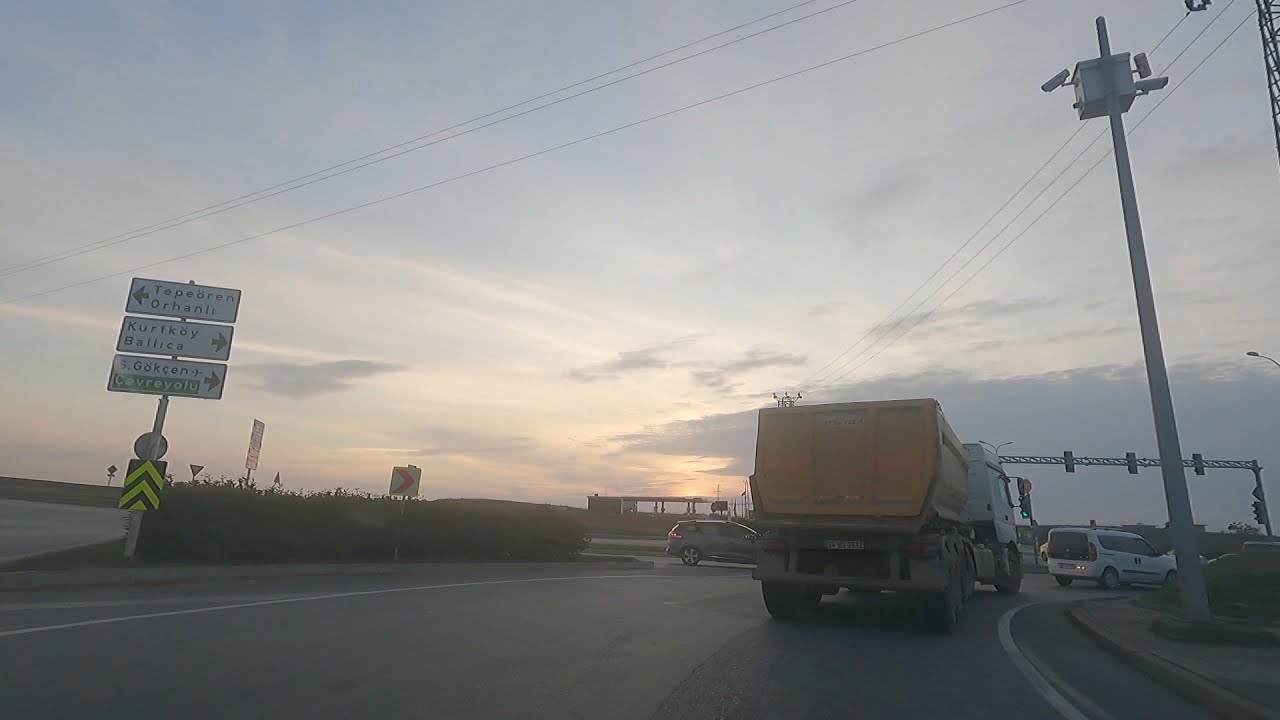From the perspective of someone driving, this image captures the moment of merging onto an intersection from inside a car. Dominating the bottom right corner, a large yellow dump truck is prominently visible, with a minivan positioned ahead of it at the front of the intersection. The gray asphalt road at the bottom of the image is framed by various street lights, traffic lights, and signs, including a metal support structure holding three stoplights. The left side of the frame features multiple signs, inscribed with text in a language other than English, including the words "Tepparan Oranji" and "Kirtki Baliks." Above, an expanse of sky occupies much of the top section, graced with power lines and clouds. The hues of the sky shift from gray to a yellowish-orange, suggesting the approach of dusk as the Sun begins to set. The scene, detailed with colors such as gray, white, yellow, black, and orange, encapsulates a typical, bustling roadway in a moment of transition.